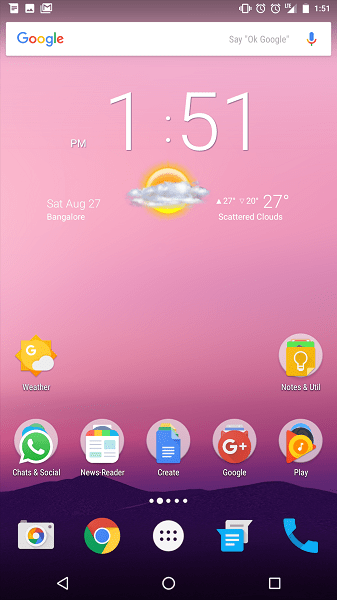A detailed screenshot of a smartphone home screen is displayed, showcasing a gradient wallpaper that transitions from a vibrant pink at the top to a deep purple at the bottom quarter of the screen. At the top of the screen, typical status icons are visible: on the left, a photo icon and a mail icon; on the right, icons for vibrate mode, two alarm clocks, LCE, signal strength, battery percentage, and the current time shown as 1:51 PM.

Directly beneath this area, a Google search bar spans the width of the screen, prominently featuring the "Google" text on the left and a microphone icon on the right. Below the search bar, the time reappears in large, bold white digits reading "1:51 PM."

Further down, the weather widget provides current weather information for Bangalore, with a graphic of the sun partially obscured by a cloud. To the left of the graphic, the date "Saturday, August 27" is displayed, while on the right, the temperature is reported as "27 degrees" with a note of "scattered clouds."

At the very bottom, a row of frequently used app icons includes Gmail, Google, text messaging, phone, and camera applications, providing quick access to these essential tools. This image encapsulates a well-organized and aesthetically pleasing home screen setup.